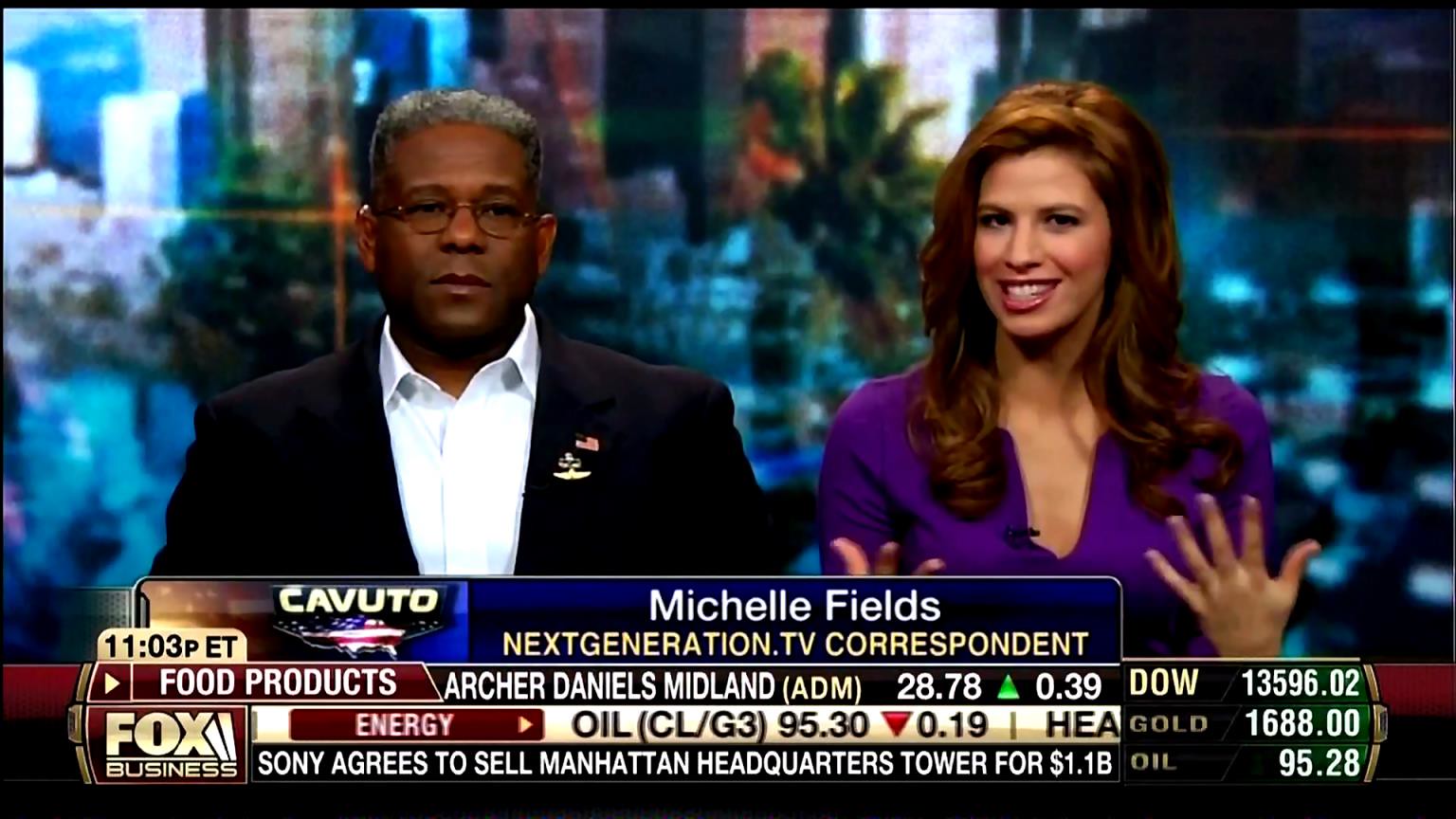This still image is taken from a Fox Business news broadcast. The frame features two individuals: an African American man on the left and a Caucasian woman on the right. The man, who has graying hair and wire-frame glasses, is dressed in a black blazer adorned with an American flag pin on the lapel over a white button-down shirt. The woman, identified as Michelle Fields, a NextGeneration.tv correspondent, has medium-length, reddish-brown hair and is wearing a purple blouse, appearing to speak with animated gestures. She also has a microphone attached to her blouse. 

At the bottom of the screen, the ticker displays various stock prices, including notable entries for the Dow, gold, and oil, and another bar reads, "Sony agrees to sell Manhattan headquarters tower for $1.1 billion." The Fox Business logo is visible on the lower left corner of the screen.